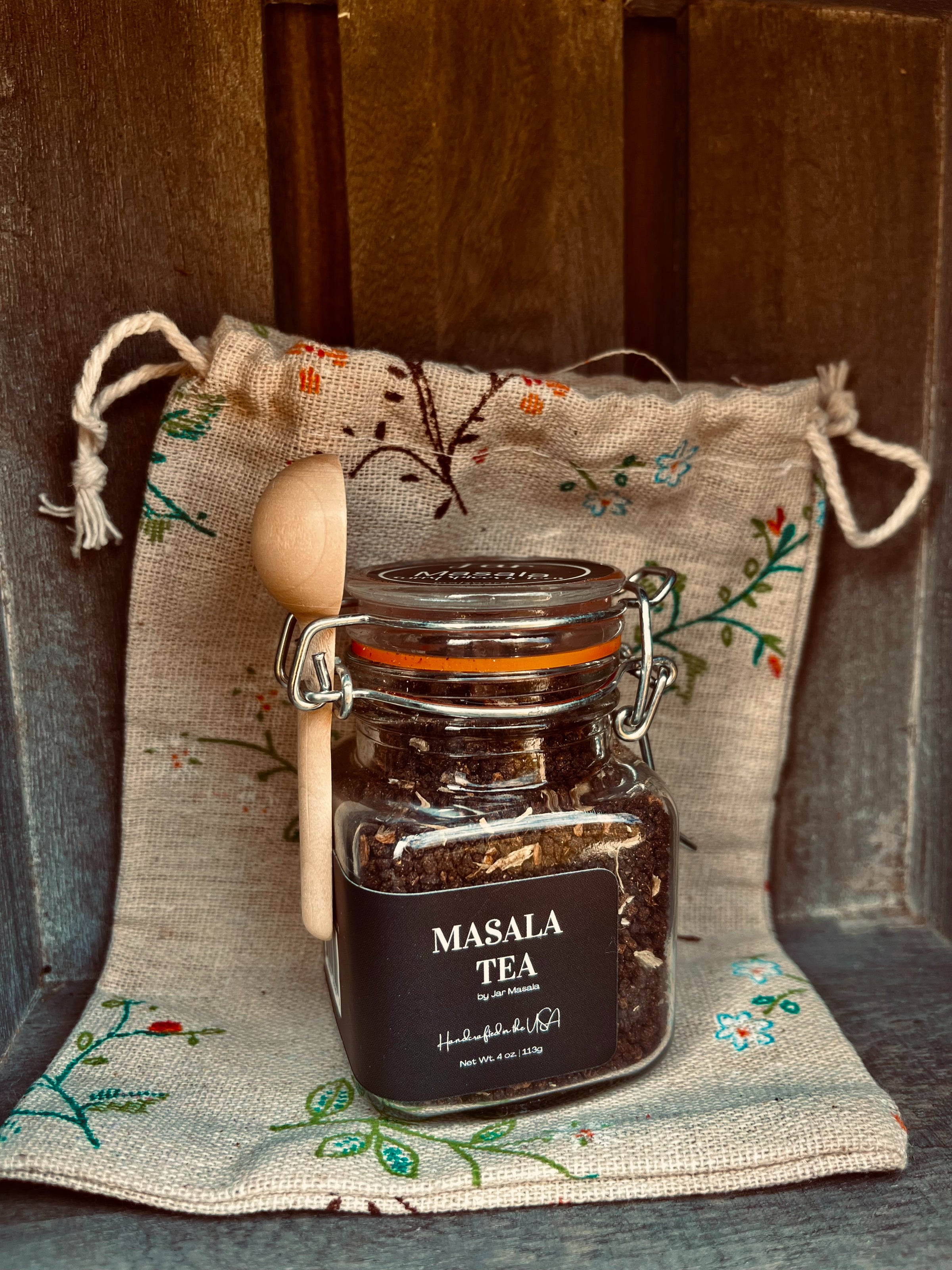The image depicts a clear glass mason jar containing tea leaves, prominently labeled with "Masala Tea" in white text on a black label, accompanied by smaller cursive and informational text. The jar features an orange sealing ring around its brim, secured by sturdy metal clamps that ensure an airtight seal. A wooden spoon is neatly tucked into a designated slot on the jar’s locking mechanism. This ensemble is situated atop a small tan burlap drawstring bag, adorned with hand-drawn images of twigs, leaves, and colorful flowers. The entire setup rests against a backdrop of wooden planks, suggestive of a rustic wooden cabinet or wall, giving the scene a cozy, kitchen-like atmosphere.